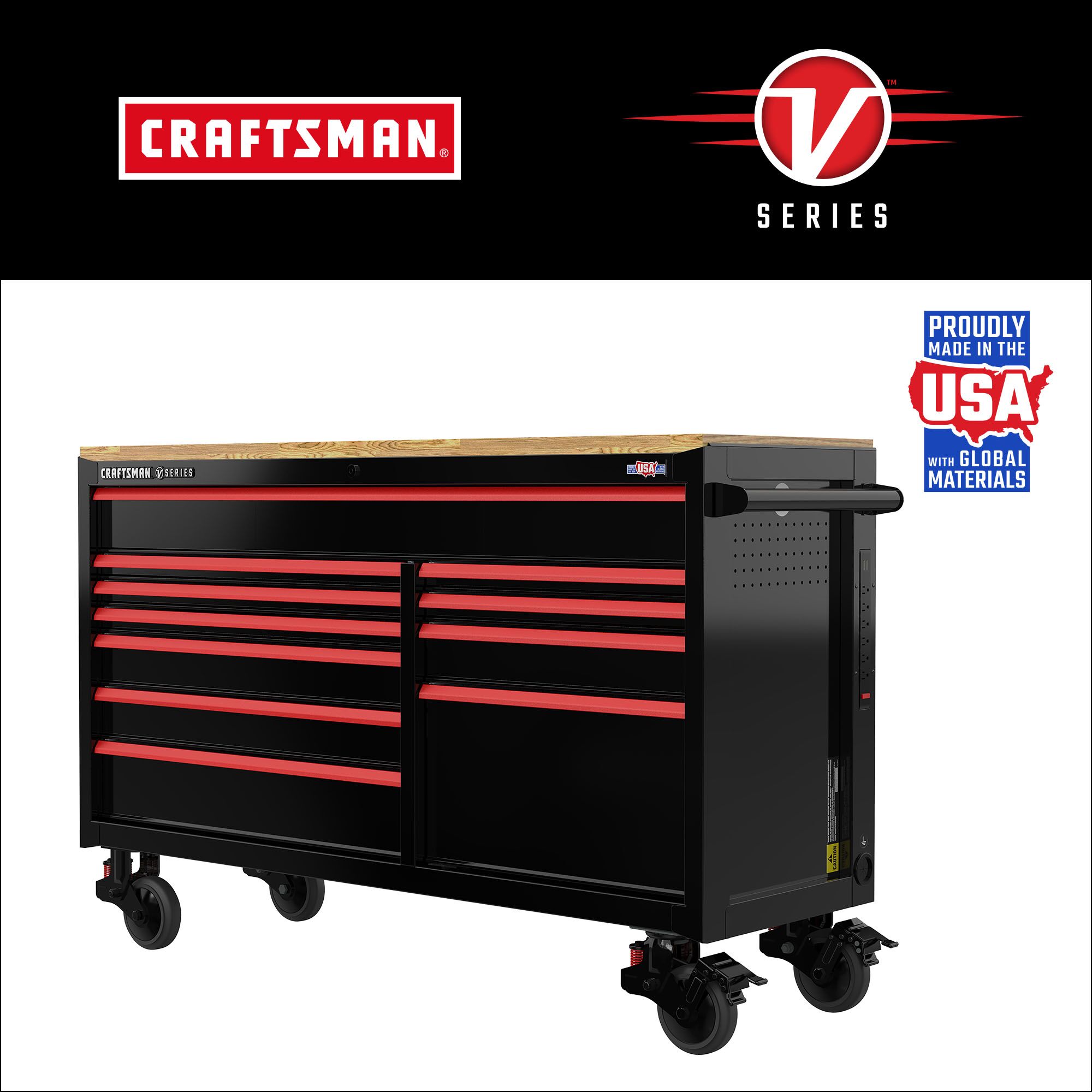This image appears to be an advertisement for a Craftsman V-Series rolling tool chest, designed for use in a shop or garage. The top section of the image has a black background, with the Craftsman logo featured in white letters inside a red rectangle with a white border on the upper left side. Adjacent to this, on the top right, is a V-Series logo showing a white 'V' inside a red circle with a white border and flanked by three red stripes. Below the logos, a stamp in red, white, and blue declares, "Proudly Made in the USA with Global Materials."

Occupying most of the image is the tool chest itself. It is predominantly black with red drawer handles and is mounted on four wheels, each equipped with a locking mechanism. The surface of the tool chest is a wooden worktop. Additionally, the chest features a convenient bar on the right side, suitable for hanging items such as a shop rag. The entire setup is showcased against a clean, white background.